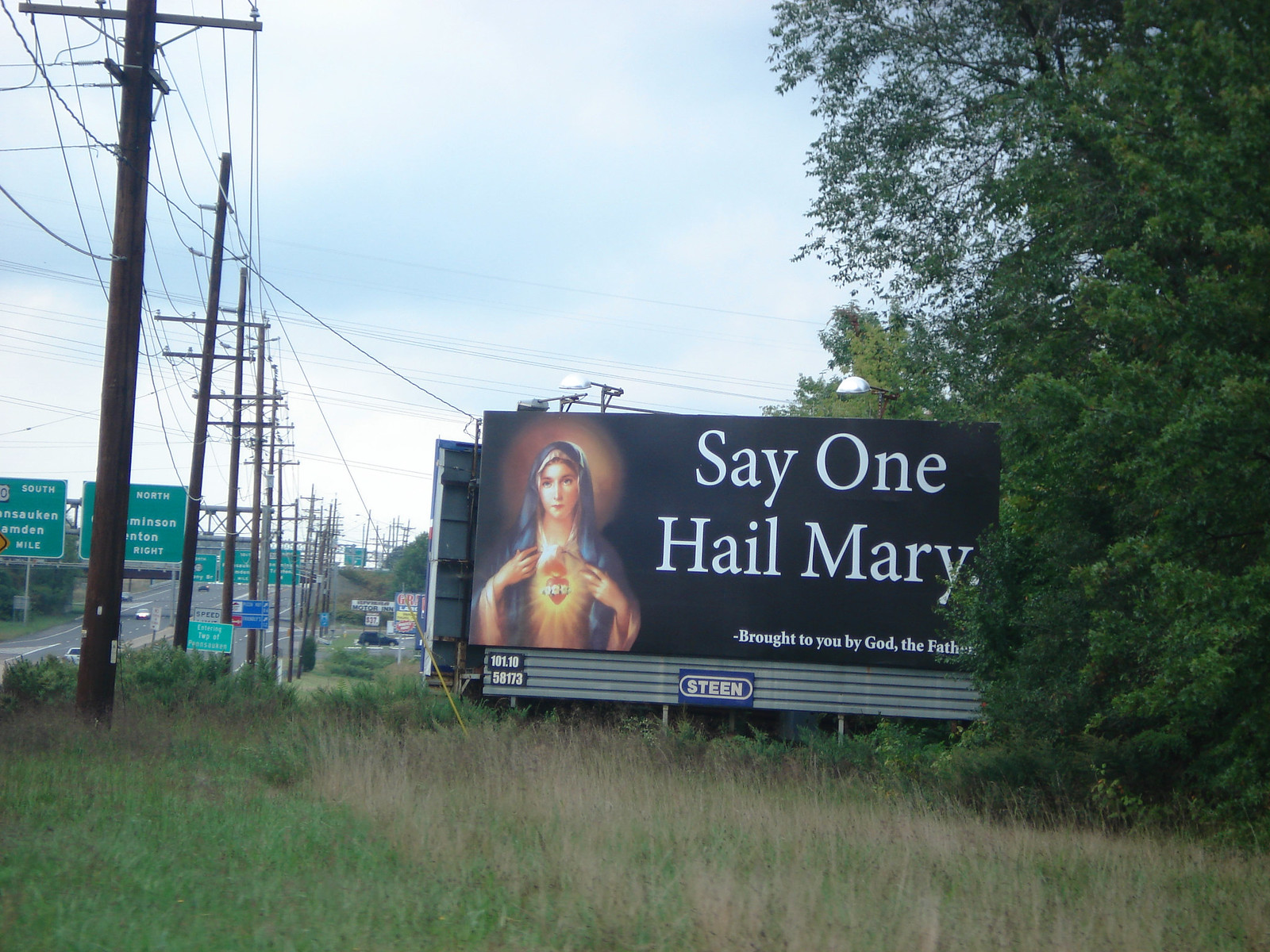The color photograph captures a scene taken from the grassy area beside a busy interstate highway during the day. Dominating the center of the image is a large, horizontal, rectangular billboard with a black background. On the left side of the billboard is a striking image of the Virgin Mary, adorned with a blue veil and a subtle halo around her head. To the right of the image, in bold white letters, the billboard reads: "Say One Hail Mary. Brought to you by God the Father." Below this, the word "Steen" is displayed on a separate blue piece of tin with a white border.

The left side of the photograph reveals a line of tall, brown electrical poles with wires stretching into the distance along the easement of the highway. This side also features large traffic signs while the right side of the image, beyond the billboard, shows several tall, leafy green trees. Background details include lights, buildings, and vehicles in motion, further emphasizing the bustling nature of the highway. The foreground consists of green and brown grasses and weeds, framing the entire scene.